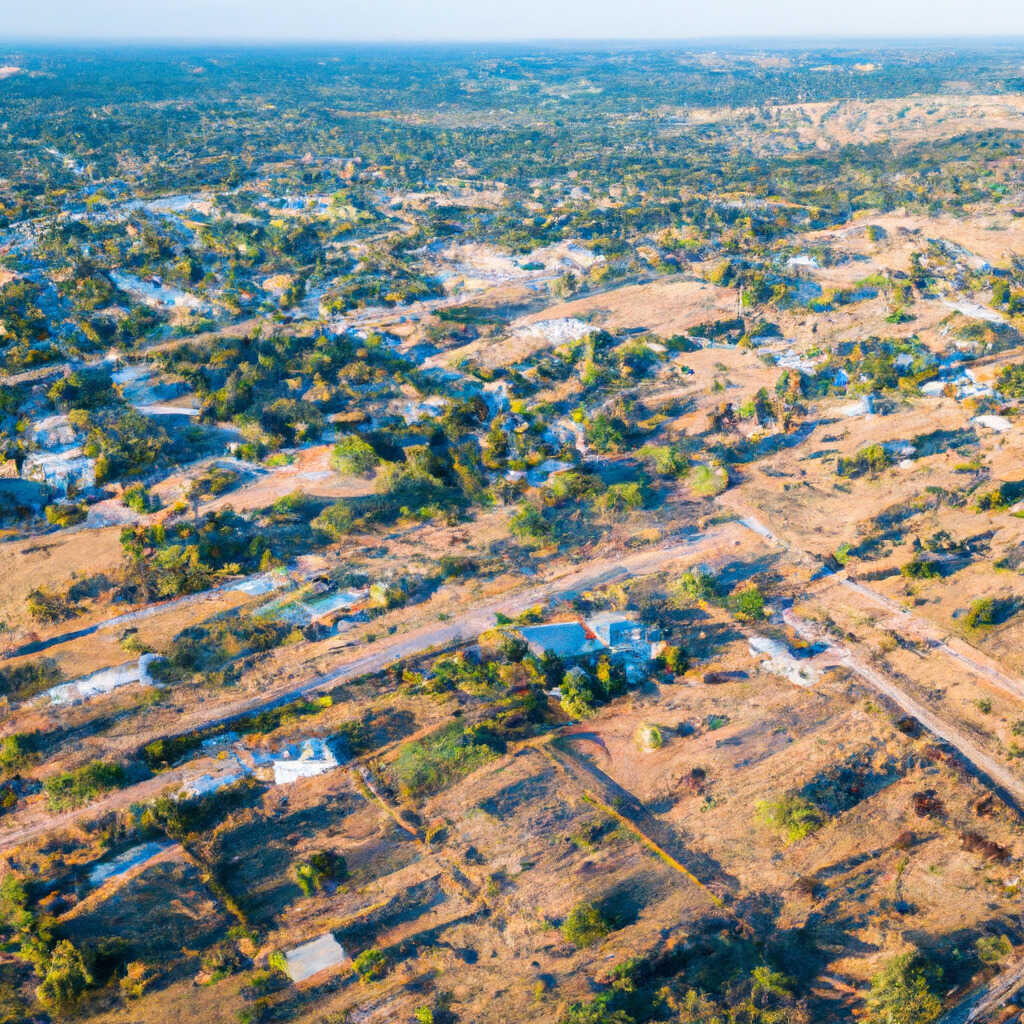This image presents an expansive, aerial view of a rural area, seemingly a painting given its somewhat smudgy and artistic texture. The scene encompasses a vast, flat landscape dotted with three farmhouses, each spaced about half a mile apart. The white farmhouse with a gray roof is prominently visible, accompanied by an asphalt driveway leading to a two-lane dirt road. The farmland around these houses showcases diverse agricultural activity; some sections are lush with gardens, while others appear freshly tilled and ready for planting. Green hedges demarcate the boundaries of different fields, contributing to the organized patchwork of the land. Sparse snow patches contrast with the predominant dirt and greenery. The image extends to a distant horizon, emphasizing the enormous expanse of this serene countryside. The skyscape, though mostly obscured, appears to have a bluish tint with hints of clouds, enhancing the calm rural atmosphere.